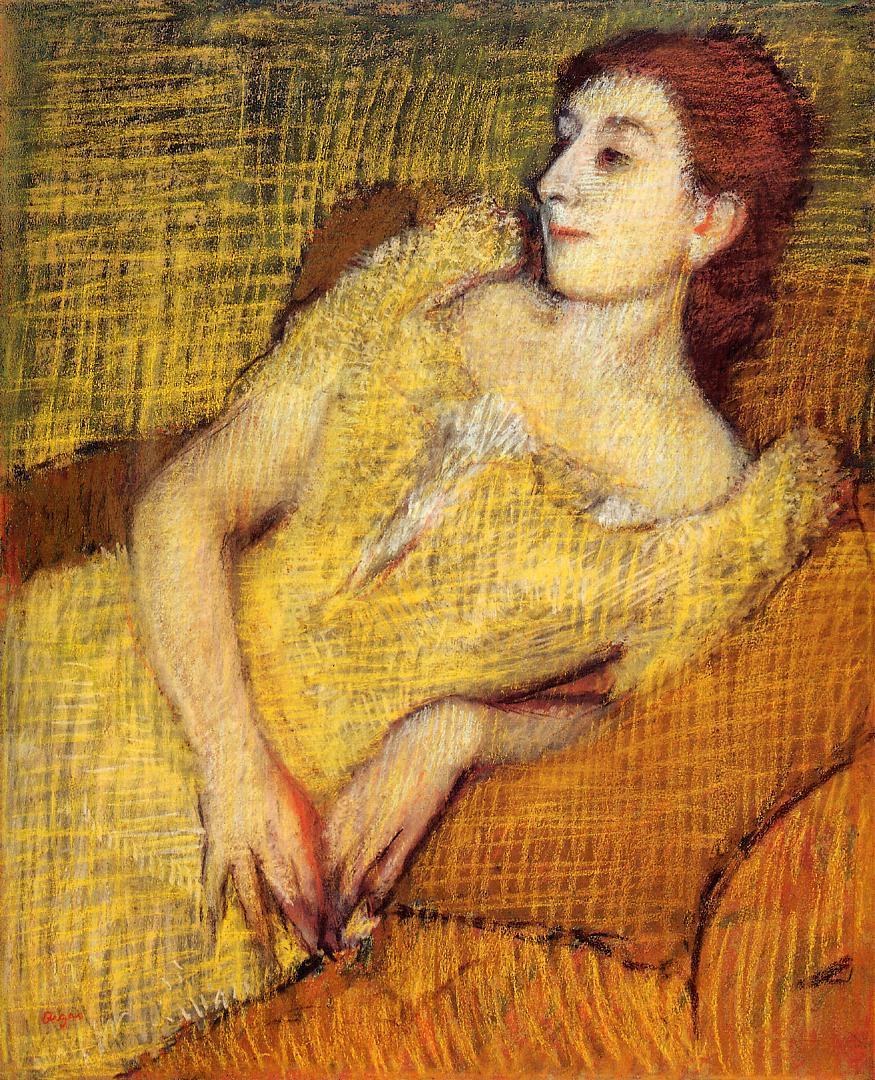The image is a detailed painting of a young woman with reddish-brown hair, reclining on her side on an orange sofa or bed, situated in front of a green-hued wall. The woman, who has a fair complexion and high eyebrows, is dressed in a yellow short-sleeve dress with some white detailing at the front. Her body faces the viewer, but her gaze is directed towards the left side. Her weight appears to be supported on her hip, with one elbow resting on an orange pillow, and her hands positioned by her left hip. The painting has an overall patchwork texture, created by yellow horizontal and vertical lines that crisscross randomly across the entire canvas. The painting is presented in portrait orientation, capturing the intimate indoor setting with a striking blend of colors and textures.